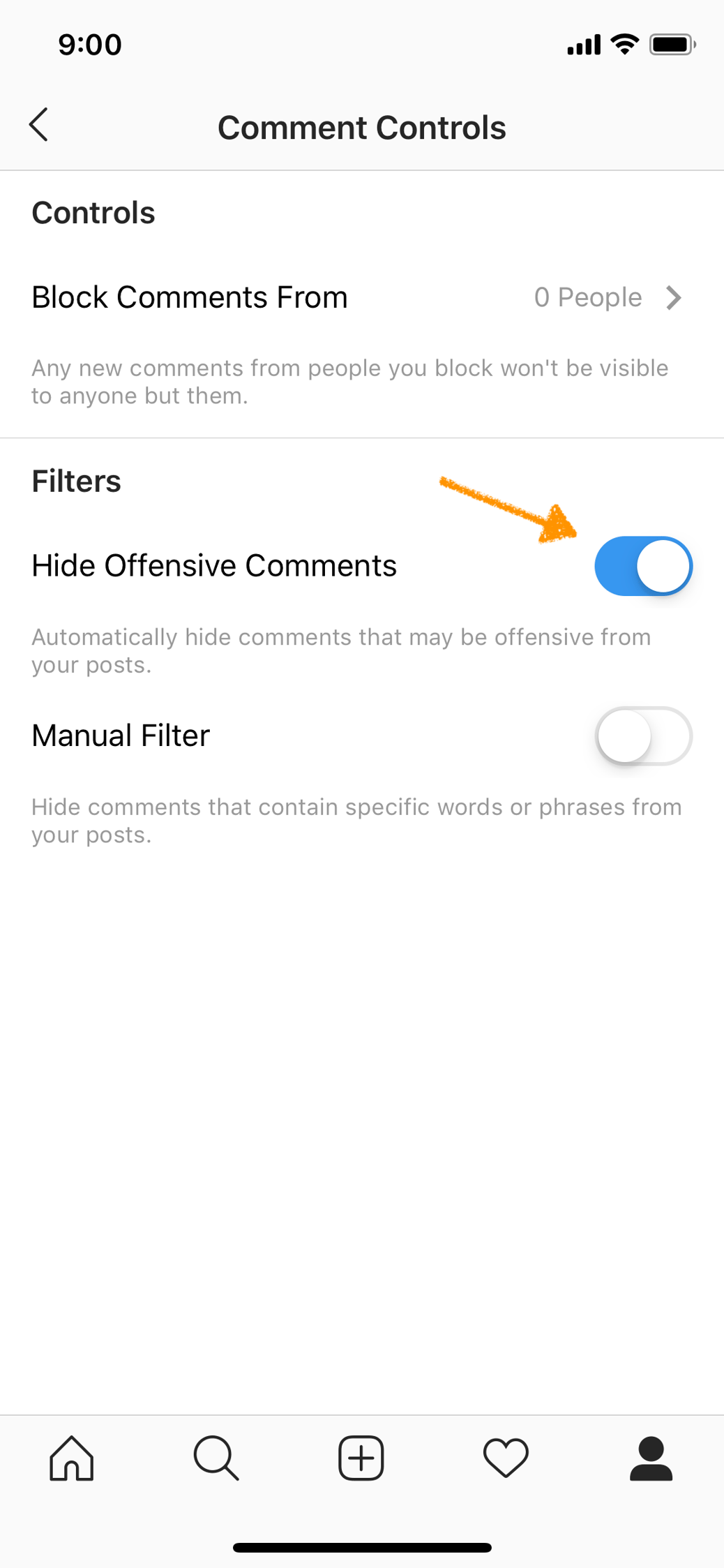The image showcases a user interface for comment control settings on a social media platform. Set against a white background, the top features a small blue box displaying "9 o'clock," accompanied by a left arrow and comment control icons.

Below, the main section presents various options under a header titled "Block Comments From," which currently indicates "zero people" and includes a right arrow for navigation. A descriptive note explains that any blocked users' comments will be visible only to them.

A thin separator line leads to the "Filters" section. Here, users can choose to "Hide Offensive Comments," with a detailed explanation and a blue toggle button currently switched on. Another filter option allows for the manual hiding of comments containing specific words or phrases, controlled by an off-position toggle switch.

The bottom of the interface displays a navigation bar in a blue box, containing icons for home, search (a magnifying glass), post creation (a square with a plus sign), likes (a heart), and user profile (a person). A thin black line runs across the bottom, demarcating the interface from the rest of the screen. The overall functionality of this interface is to enable users to manage and hide offensive comments, enhancing their control over interactions on their posts.